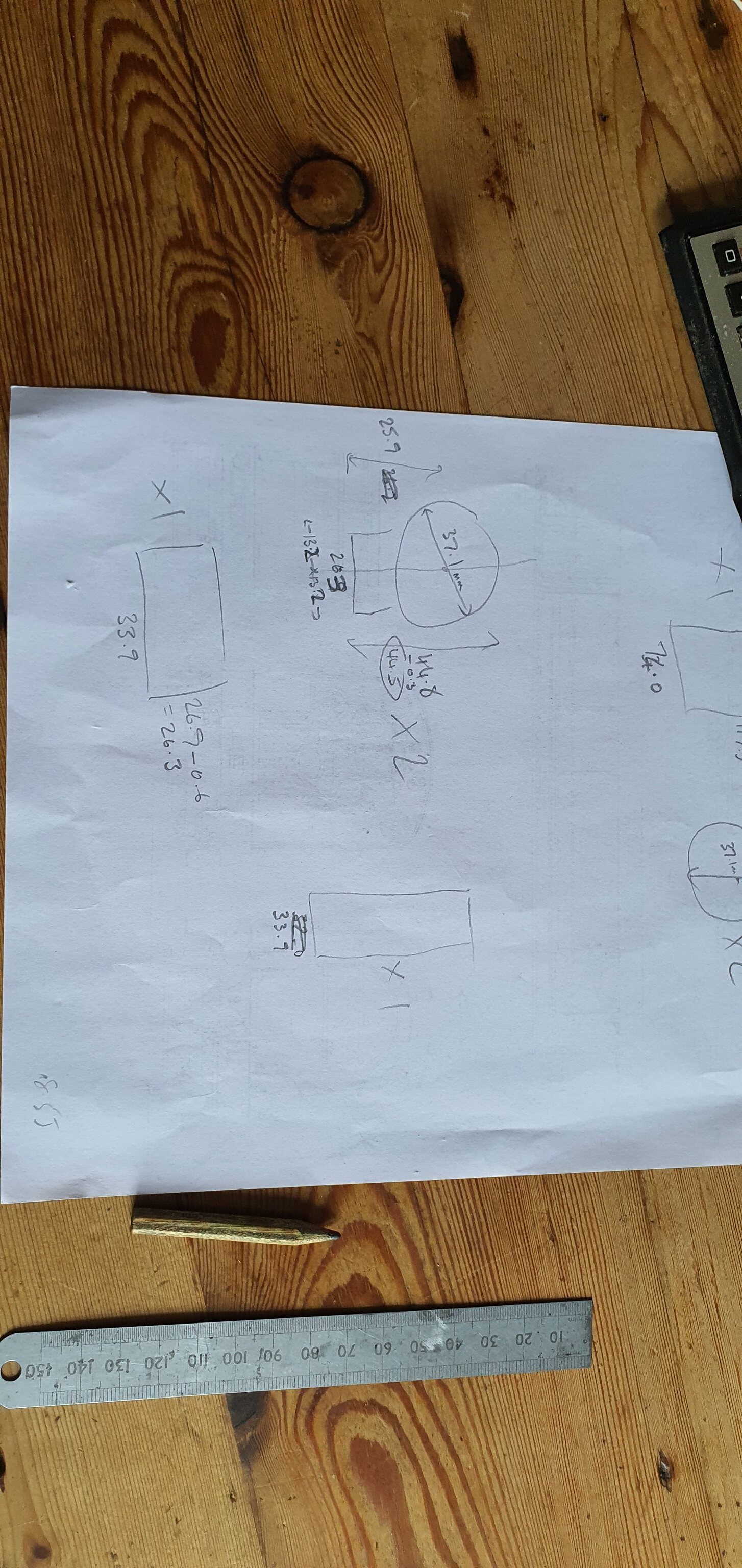The image features a piece of paper resting on a wooden table near the bottom of the frame. Positioned diagonally on the paper, a vintage metal ruler showcases its centimeter and millimeter markings. Between the ruler and the paper lies a well-worn, half-length pencil. 

The paper itself contains a variety of graphs and mathematical notations. Positioned sidelong on the screen, the numerical and geometric details are clear. On the bottom left of the paper, there's a rectangle annotated with "33.9" at the bottom edge and "26.9 - 0.6 = 26.3" on the right edge. A "×1" is marked on the left side of this rectangle. 

Above the rectangle, a circle is labeled "37.1 millimeters in diameter," accompanied by some formulas on its side. Near the top of the page, which is slightly cut off, a square is marked "74.0" at the bottom edge and has a "×1" notation nearby. To the right of this square, another circle with a diameter of "37.1" is noted, along with a "×2" indication. Below this is a long rectangle labeled with "×1" next to it and "33.9" on the bottom side. The document appears to depict technical or engineering calculations.